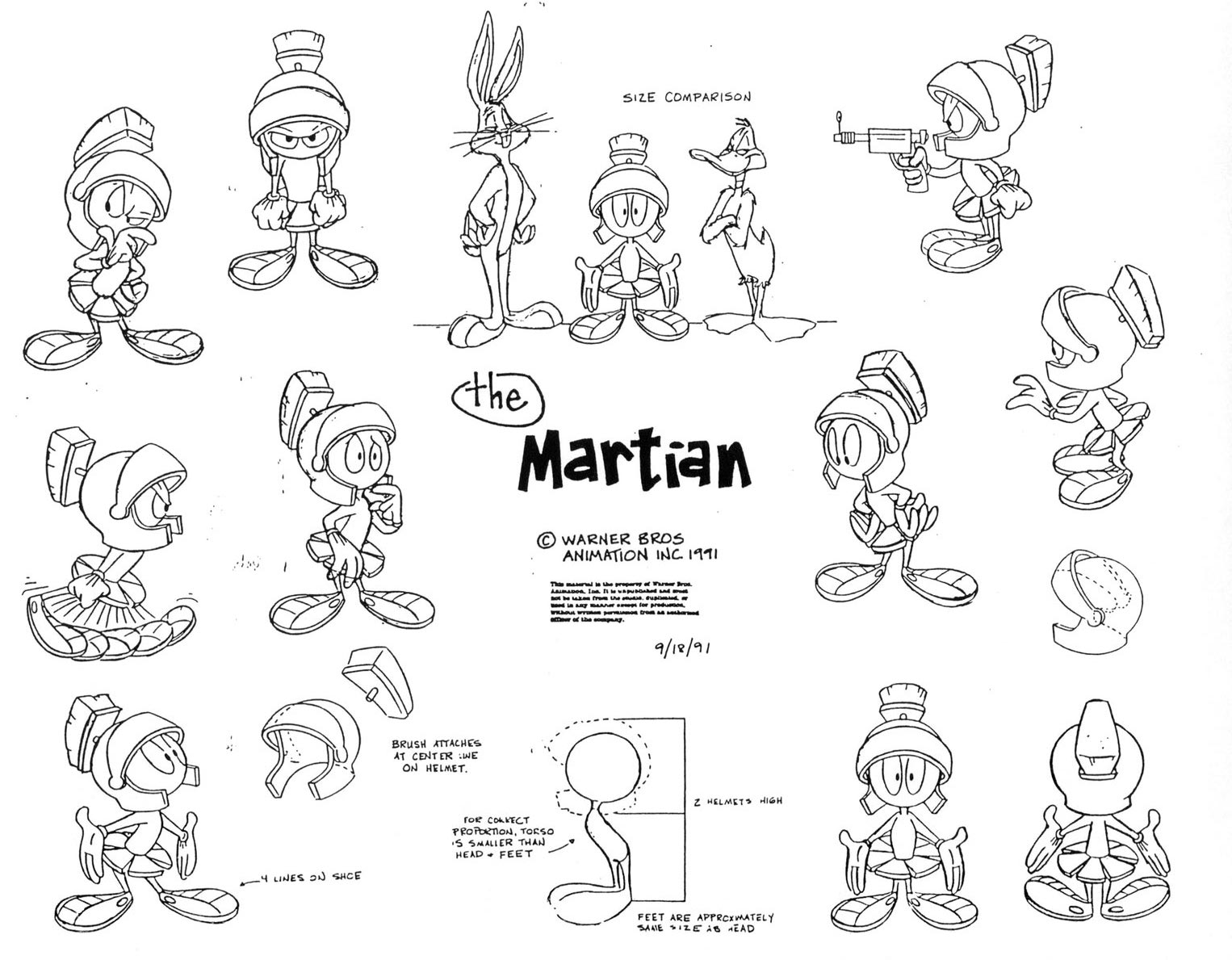The image is a detailed, black-and-white sketch sheet from Warner Brothers Animation Inc., dated 1991 and marked with the number 91891. At the top, it says "size comparison" and showcases several cartoon characters, prominently featuring Marvin the Martian in various poses and views. The words "The Martian" are boldly written in the center of the sheet. Surrounding Marvin are sketches of other Warner Brothers characters, including Bugs Bunny and Daffy Duck. Marvin is depicted in different action poses: standing, running, and shooting a laser gun. There's also a detailed diagram labeling aspects of Marvin, with notes indicating details such as "feet are approximately the same size as head" and "Brush Attaches." At one point, Marvin's helmet is depicted separately, with a note about unhelmeting. The sheet provides a comprehensive view of Marvin the Martian from multiple angles and includes annotations, suggesting how the character should be depicted and animated.